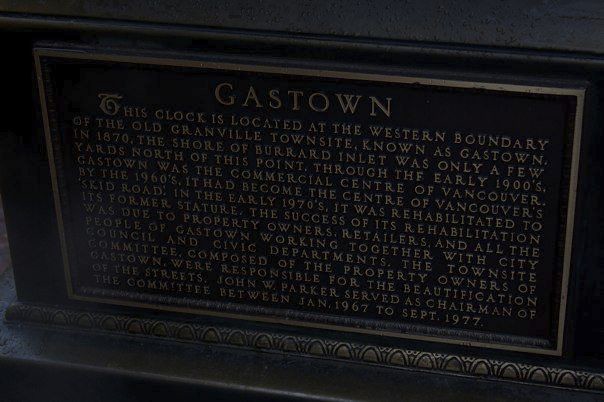This image showcases a plaque with a black background and a gold border, displaying gold lettering. The plaque, likely mounted indoors on a wall, bears the heading "Gastown." It provides a detailed historical account of Gastown, starting with its location at the western boundary of the old Granville town site. The plaque mentions that in 1870, the shore of Burrard Inlet was just a few yards north of this point. It highlights Gastown's evolution from being Vancouver's commercial center in the early 1900s to becoming the heart of the city's Skid Road by the 1960s. The narrative continues, describing the area's rehabilitation in the early 1970s, which restored its former prestige. This revitalization was attributed to the collaborative efforts of property owners, retailers, the city council, and civic departments. A town site committee, led by John W. Parker from January 1967 to September 1977, played a crucial role in beautifying the streets of Gastown. The clock mentioned in the plaque serves as a historical landmark, emphasizing Gastown's significant role in Vancouver's history.